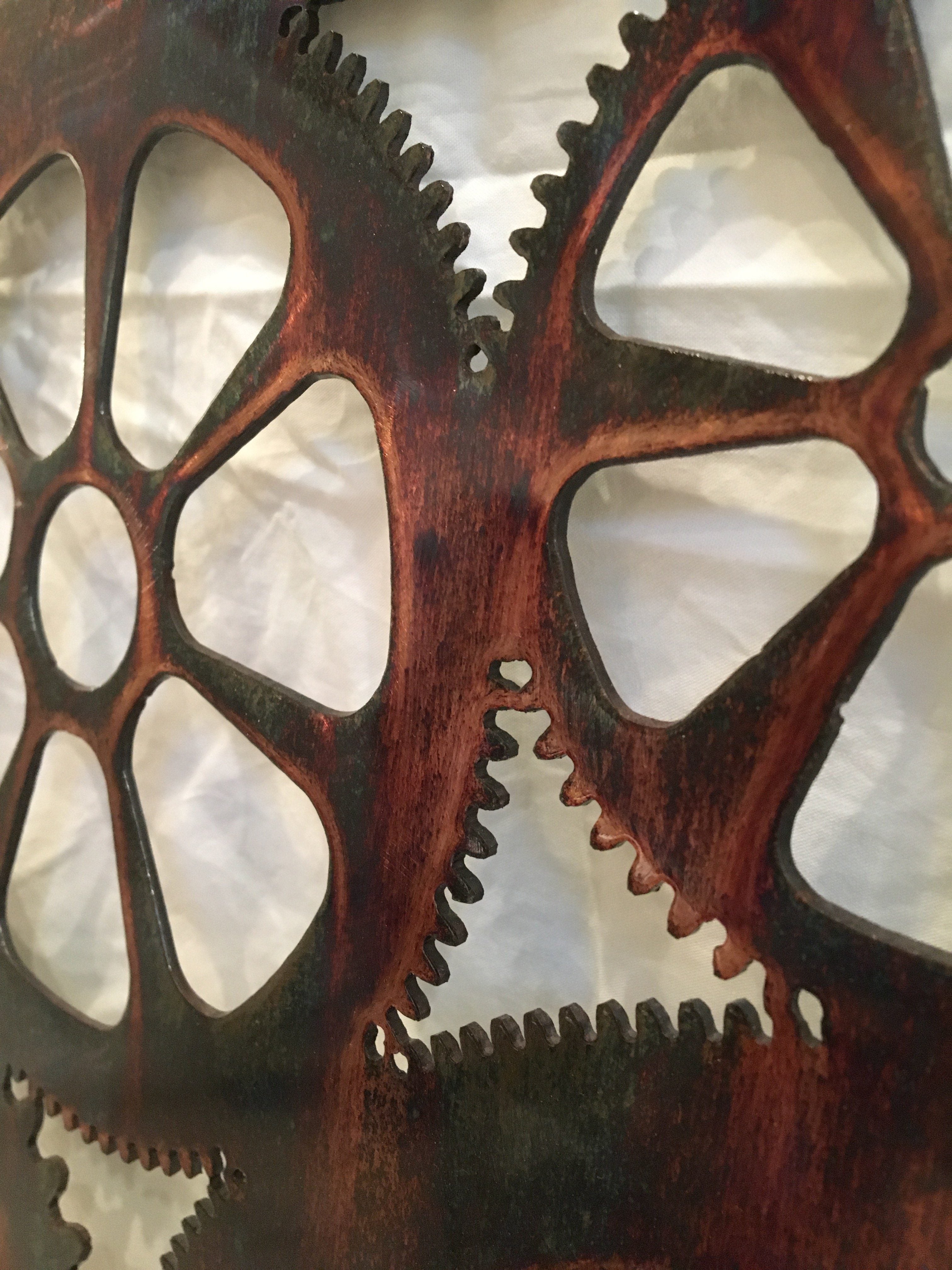The image depicts a detailed wooden sculpture resembling interconnected gears. Crafted to appear as a single cohesive piece, the gears are fused together, suggesting a non-functional, artistic representation rather than actual mechanical parts. The wood, potentially redwood or mahogany, has been meticulously finished with varnish or lacquer, giving it a polished appearance. The dark brown hue of the wood, accentuated by noticeable grain patterns, indicates a carefully stained surface that shows signs of wear from frequent handling. The backdrop is a plain white cloth, its folds and wrinkles casting subtle shadows, with no additional context to determine the sculpture's size. The minimalist setting and the intricate design converge to highlight the artistic ingenuity and craftsmanship of the piece.